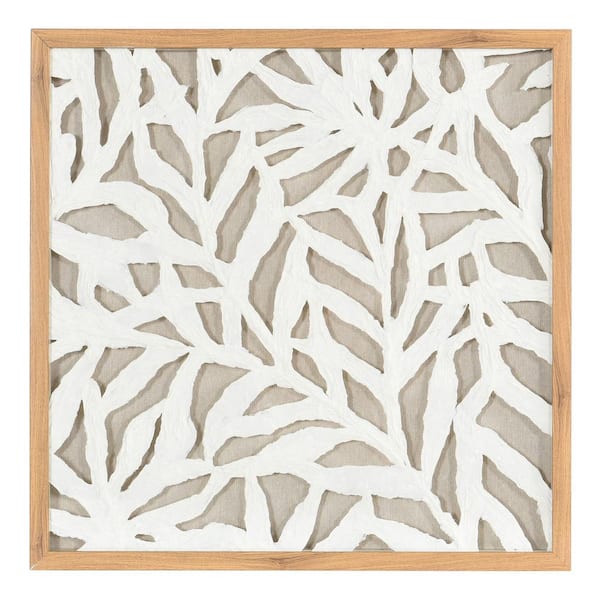The image is a detailed piece of artwork set in a thin, light brown wooden frame that forms a perfect square. Centrally positioned against a white surface, the artwork appears to play with dimensions, giving off the impression of being either a computer-generated design, a painting, or an intricate paper cutout. The dominant colors are white, beige-tan, and various shades of gray. The artwork consists mainly of jagged gray shapes or shards, reminiscent of broken glass, with subtle linear patterns resembling leaves or weaves throughout. These lines create a slightly embossed or 3D effect, adding depth to the composition. Despite its understated and drab appearance, with no discernible text or standout images, the piece showcases the finesse of intricate cutouts and the minimalist aesthetic of modern art.